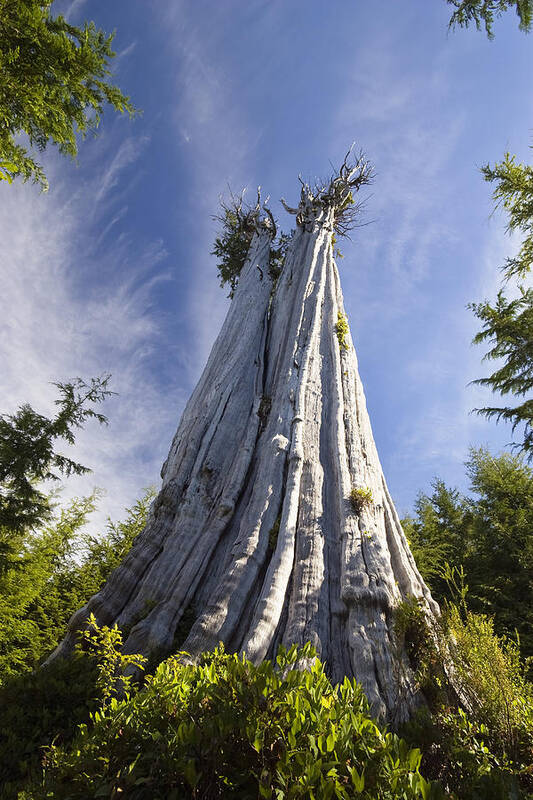The photograph portrays a towering, ash-colored remnant of what was once a majestic sequoia or redwood tree, located in Olympic National Park, Washington, U.S. The image, taken from the base and looking straight up, emphasizes the imposing height of the stump, which stretches tens of feet into the sky. The driftwood-gray surface of the tree is largely bare, revealing intricate bark lines, except for the top, where sparse, stunted branches show signs of greenery, hinting at a vestigial resurgence of life. Surrounding the base of the stump are lush bushes and the leaning tops of conifer trees, enhancing the scene's tranquility. The background features a strikingly blue sky interspersed with fuzzy, stringy clouds, which, along with the sunny rays illuminating the tree, contribute to a serene and visually stunning composition.